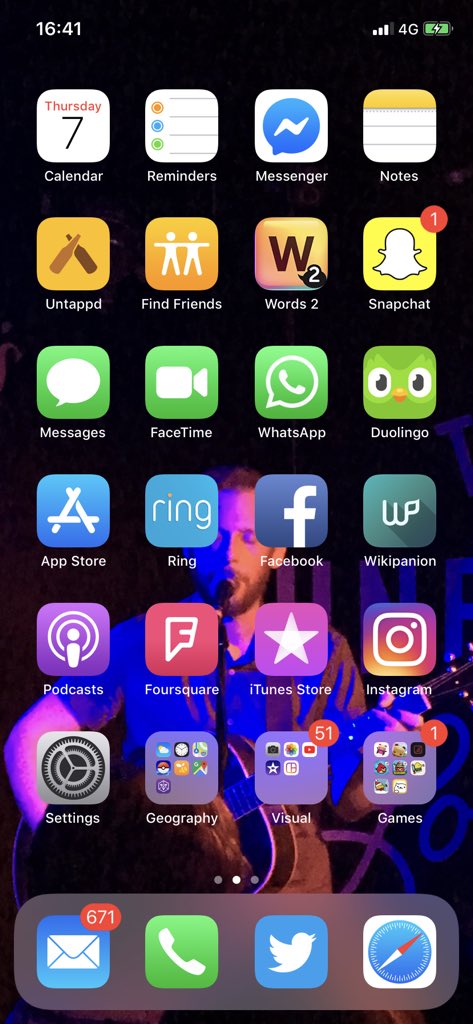This phone screenshot features a dynamic background image of a musician passionately playing guitar on a stage illuminated with vibrant blue and red lights. The main screen showcases an array of app icons neatly arranged. Dominating the screen are various apps, including Calendar, Reminders, Messenger, Notes, Untappd, Find Friends, Words, Snapchat, Messages, FaceTime, WhatsApp, Duolingo, App Store, Ring, Facebook, Wikipanion, Podcasts, Foursquare, iTunes Store, Instagram, and Settings. Additionally, there are app groupings labeled Geography, Visual, and Games.

At the bottom, the classic navigation bar displays essential apps: Messages, Email, Phone, Twitter, and Safari browser. The current time reads 16:41 (4:41 PM), and the phone is actively charging. Each app retains its distinct iconography: Duolingo's green owl, WhatsApp's green chat bubble, Messages’ green chat bubble, FaceTime’s camera icon, Snapchat’s yellow box with a white ghost, Messenger’s blue chat bubble with a white lightning bolt, and Twitter’s blue square with a white bird, among others. This well-organized and visually appealing phone layout reflects a user familiar with diverse digital tools.